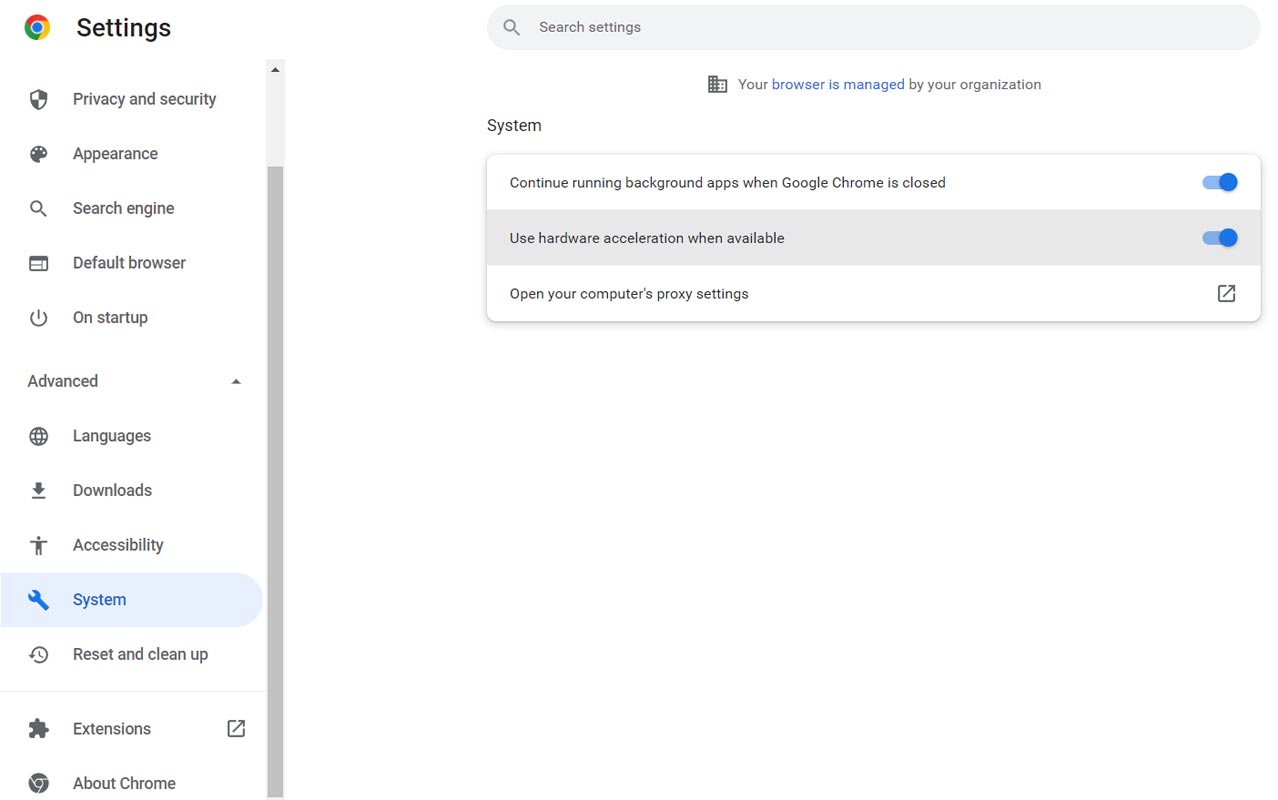In the image, we see the Google Chrome settings page featuring a detailed layout of various options and icons. At the top left, there is the Google Chrome logo followed by the "Settings" header. Below this is a vertical menu that includes a range of settings categories, each accompanied by a specific icon. 

The first category is "Privacy and Security," represented by a shield icon. Next is "Appearance," depicted with a paint palette icon. The "Search Engine" option is marked by a magnifying glass icon, while "Default Browser" is symbolized by a browser icon. The "On Startup" category features a power symbol.

Continuing down the menu, the "Advanced" section is indicated by an upward-pointing arrow. This expands to include additional settings such as "Languages" with a globe icon, "Downloads" with a downward arrow and line icon, "Accessibility" with a person icon, "System" with a wrench icon, and "Reset and Cleanup" marked with an arrow circling around a dash, resembling a clock.

Further down, the "Extensions" category features a puzzle piece icon, paired with a box and arrow icon on the right pointing diagonally outward, suggesting more options. The "About Chrome" section is denoted by the Chrome symbol.

To the right of the Chrome logo and "Settings" header at the top, there is a search bar with a magnifying glass icon and the text "Search settings." Underneath this bar, it states "Your browser is managed by your organization."

Beneath the menu and central header, we see a "System" category with a blue-striped box that covers specific system settings. The settings listed here include "Continue running background apps when Google Chrome is closed," which has an enabled blue slider, and "Use hardware acceleration when available," also enabled with a blue slider. Lastly, there is an option to "Open your computer's proxy settings" accompanied by the same box and arrow icon pointing diagonally out to the right.